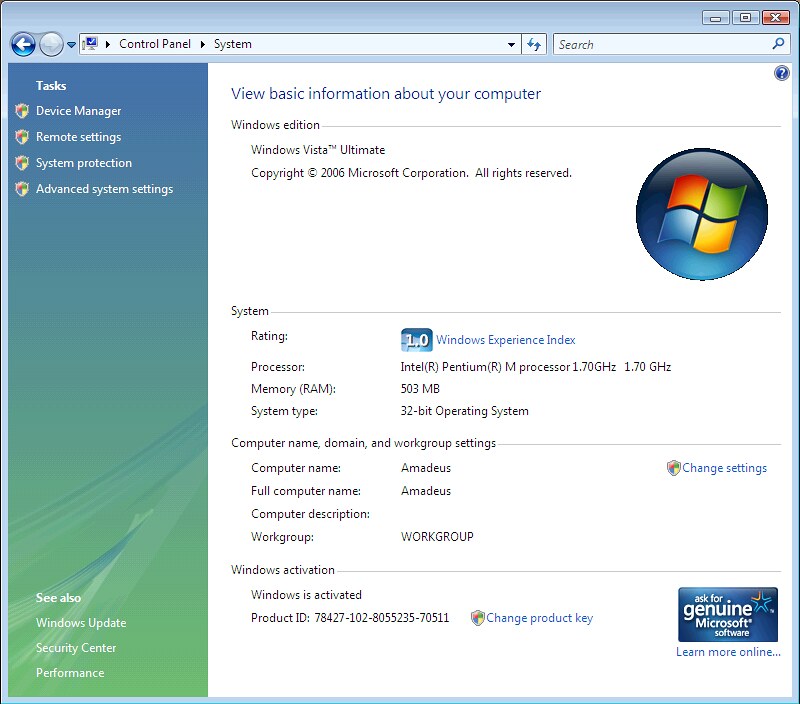This detailed color image is a screen capture from the Control Panel of a Windows Vista Ultimate computer. At the top of the screen, it reads "Control Panel" with an arrow pointing to "System." On the left sidebar, which transitions from blue to yellowish, there are options listed: Tasks, Device Manager, Remote Settings, System Protection, and Advanced System Settings. The main part of the display is predominantly white and features the header "View Basic Information about your computer." 

This section includes details such as:
- **Windows Edition:** Windows Vista Ultimate, Copyright 2006 Microsoft Corporation.
- A large circular Windows logo in blue.
- **System Rating:** 1.0, Windows Experience Index.
- **Processor:** Intel Pentium Processor 1.70 GHz.
- **Memory (RAM):** 503 MB.
- **System Type:** 32-bit Operating System.
- **Computer Name:** Amadeus.
- **Workgroup:** WORKGROUP (in all caps).
- **Windows Activation:** "Windows is activated" followed by Product ID: 78427-102-8055235-70511.

This screen provides a comprehensive overview of the system's basic properties and specifications, typical for the Control Panel on any Windows computer.